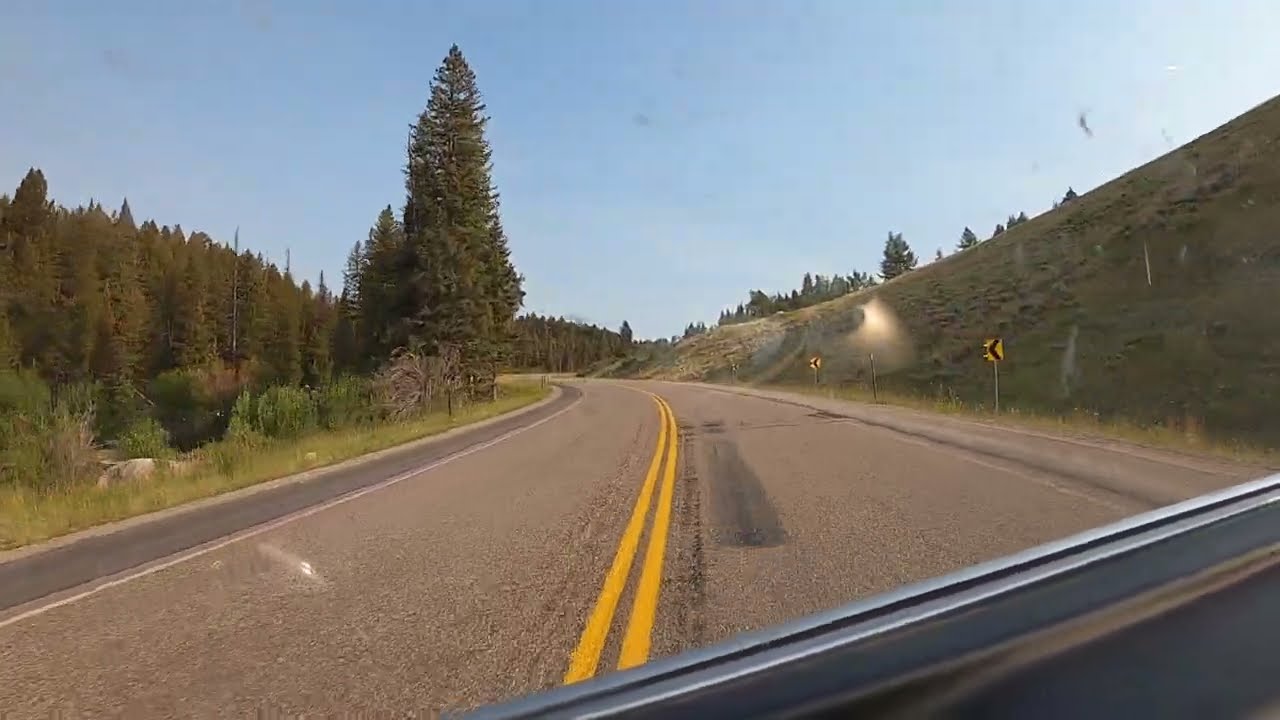The photograph, taken from inside a car, depicts a two-lane road set against a natural backdrop. The road, characterized by its double yellow dividing lines, begins from the bottom of the image and gently curves to the left before veering sharply right behind a grassy hill. On the right-hand side, two rectangular yellow street signs with black arrows warn of upcoming curves, set against the grassy hill. The left-hand side features a strip of green grass leading down to a river, beyond which a dense tree line extends out of view. Several larger trees, including a prominent pine tree, mark the edge of the curve. The sky above is mostly clear, a rich blue on the left transitioning to a brighter, whitish hue on the right, suggesting the sun’s position. The scene is devoid of humans and animals, immersing the viewer in a vividly colored landscape of greens, yellows, and the grayscale of asphalt.